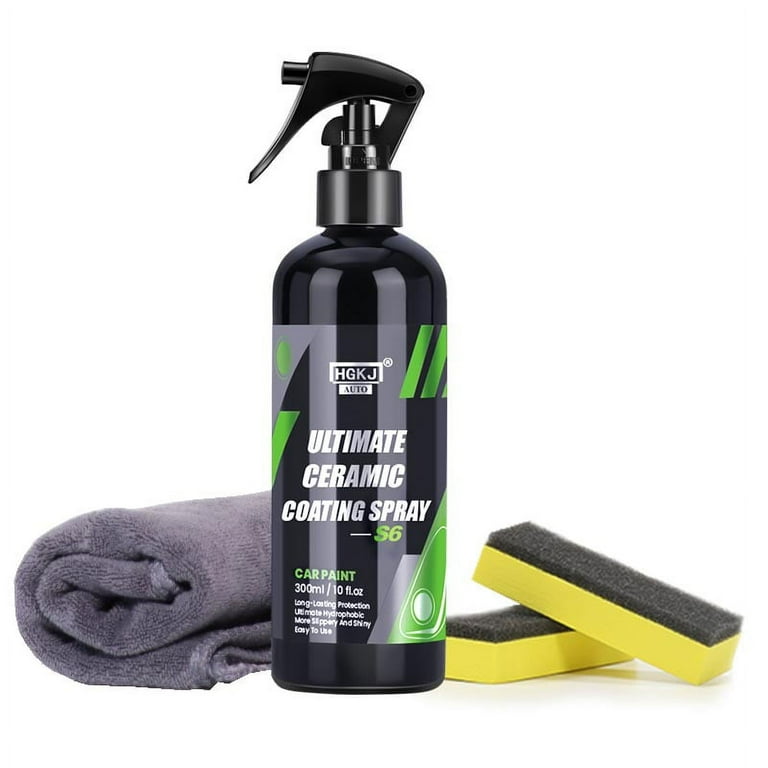This is a detailed close-up photograph of a black spray bottle labeled as "HGKJ Auto Ultimate Ceramic Coating Spray." The bottle features a black cap and sprayer, with text in various colors and designs. The brand name is presented within a gray rectangle on a black background, and the label reads "Ultimate Ceramic Coating Spray" in silver, followed by "S6" in green. Near the bottom, green text states "Car Paint," and additional silver text notes "300 milliliters / 10 fluid ounces," along with descriptions such as "Long-Lasting Protection," "Ultimate Hydrophobic," "More Slippery and Shiny," and "Easy to Use." The bottle also has green decorative elements throughout the design. Positioned to the left of the bottle is a curled-up gray microfiber towel, and to the right are two sponges with yellow bases and black tops, indicating different sponge textures. The entire set is displayed against a white background.